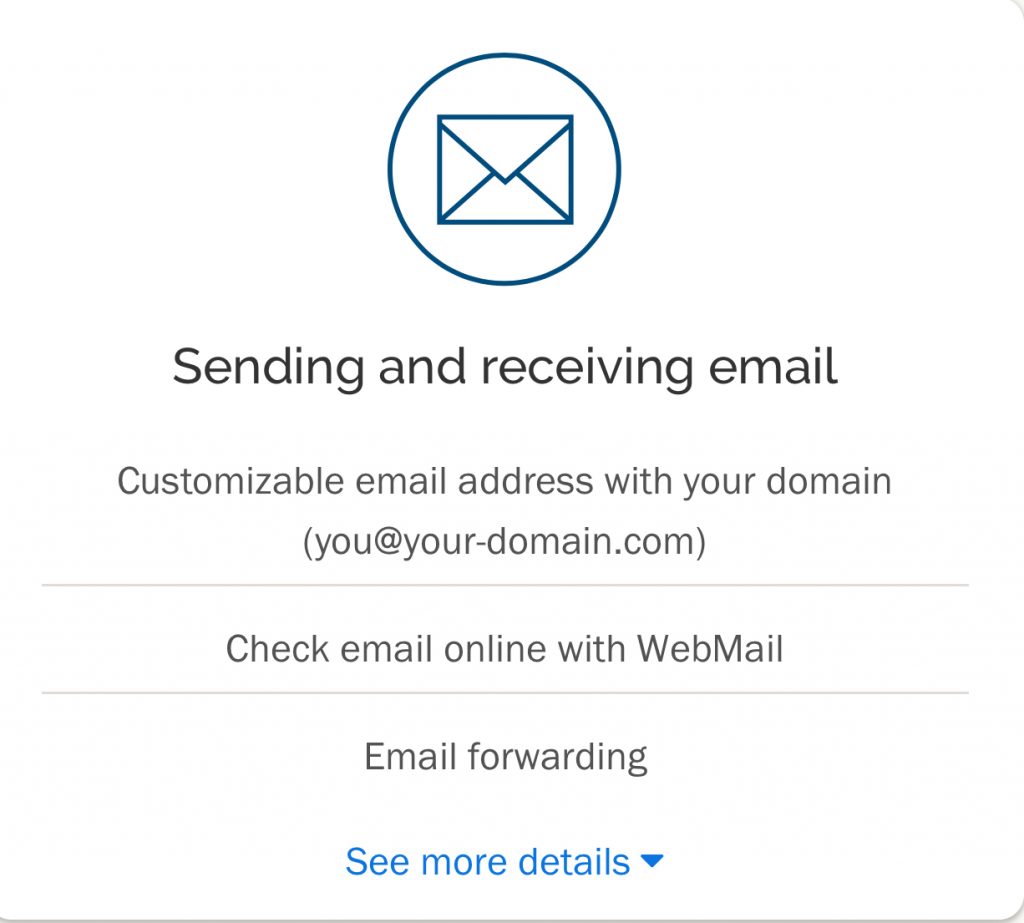The image features a white background with predominantly black text and some blue elements. At the top center, there is a dark blue circle with a white interior, inside of which is a dark blue envelope icon, also filled with white. Below this icon, the text reads "Sending and Receiving Email." Following this, the message continues, "Customizable email address with your domain. You@yourdomain.com." Further down, it states, "Check email online with webmail," and then "Email forwarding." At the very bottom, there is a blue drop-down menu that reads "See more details."